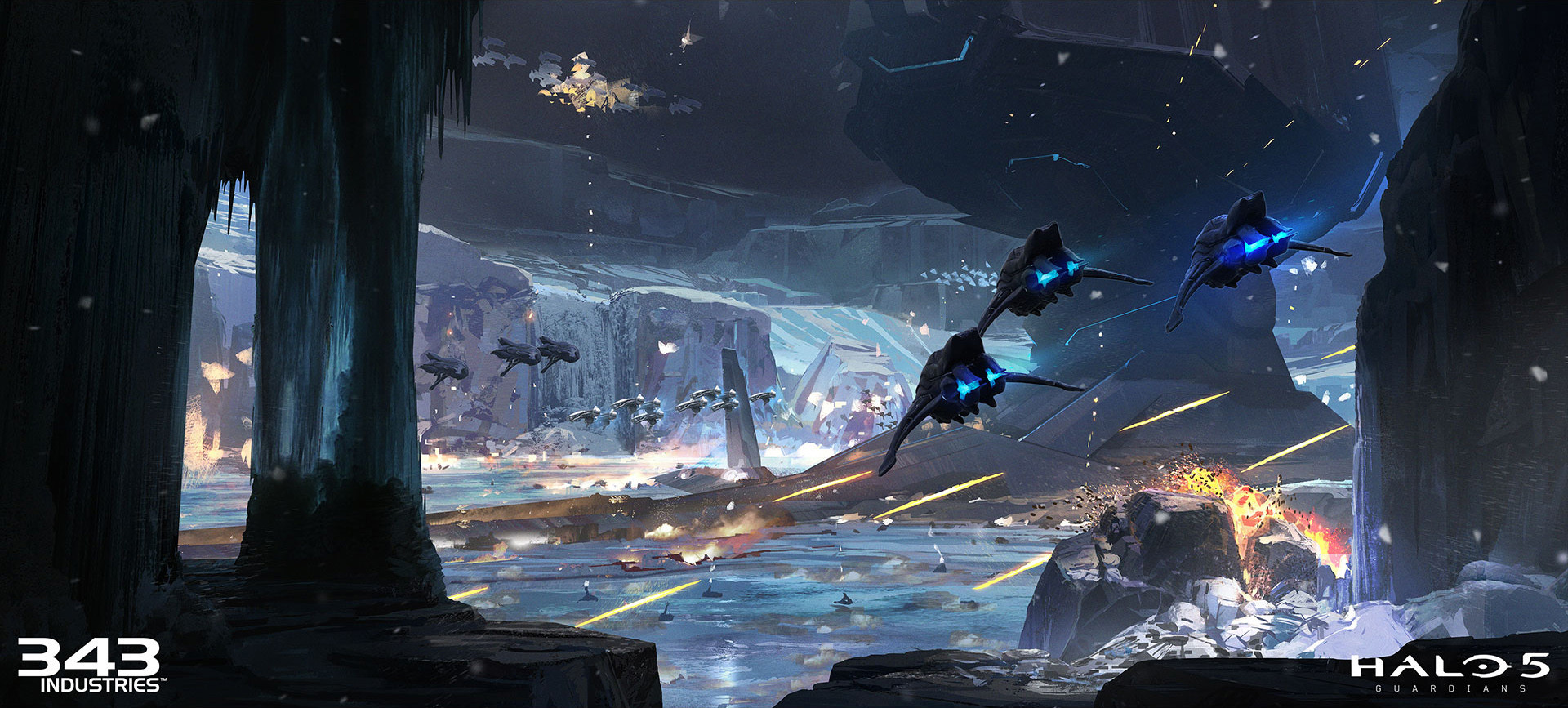This wide-angle screenshot from the video game Halo 5: Guardians presents an intense, futuristic battle scene set in a vast, gray canyon, potentially with icy surfaces. Three identical black warships, leaving blue jet trails from their engines, fly in close formation, maneuvering diagonally to evade an onslaught of laser beams and fiery projectiles. The sky is filled with numerous laser bullets and vibrant explosions that cast hues of orange and yellow across the predominantly blue-toned scene. Amidst the hovering spacecraft, a centerpiece yellow floating city and various other structures dot the background, adding to the chaotic battlefield. In the bottom corners, "343 Industries" is inscribed in white on the left, while "Halo 5: Guardians" appears on the right, anchoring this image in the iconic Halo universe.